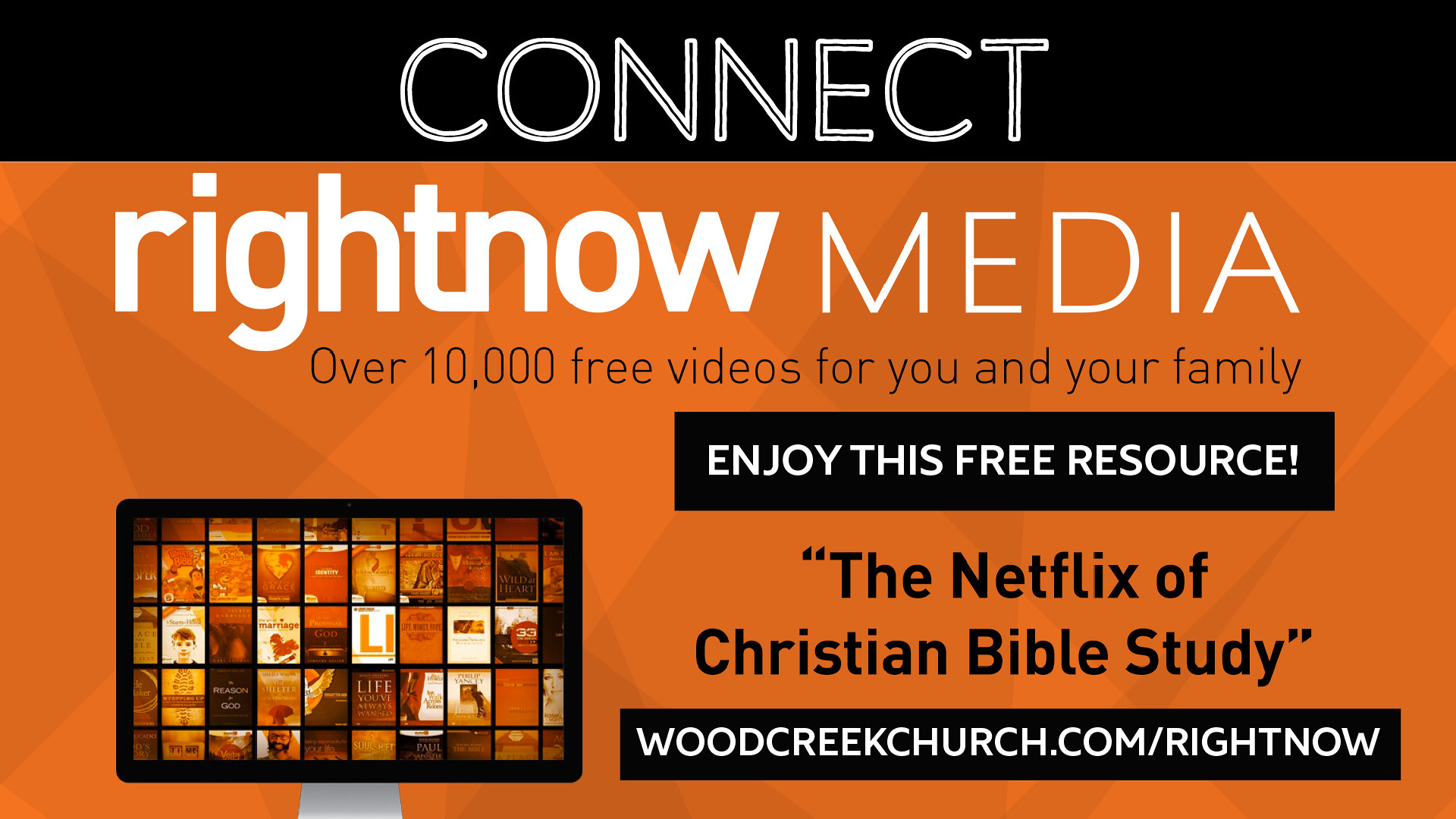The image is a detailed advertisement primarily in black and orange hues, highlighting the  benefits of the service. At the top, the ad features a black bar with the word "Connect" prominently displayed in white text. Below this, a bold orange background showcases the white text "Right Now Media." Following this, the ad states in black text, "Over 10,000 Free Videos for You and Your Family." Further down, there is a black box containing the message "Enjoy This Free Resource" in white text, accompanied by a descriptor in black text below: "(The Netflix of Christian Bible Study)." Another black box at the bottom provides the web address "woodcreekchurch.com/rightnow" in white text. In the bottom left corner, a color image of a large flat-screen TV is depicted, showing a grid of various colorful content thumbnails, resembling books or movie covers. The TV sits on a sleek silver stand, with shadows and black trim accentuating the screen.